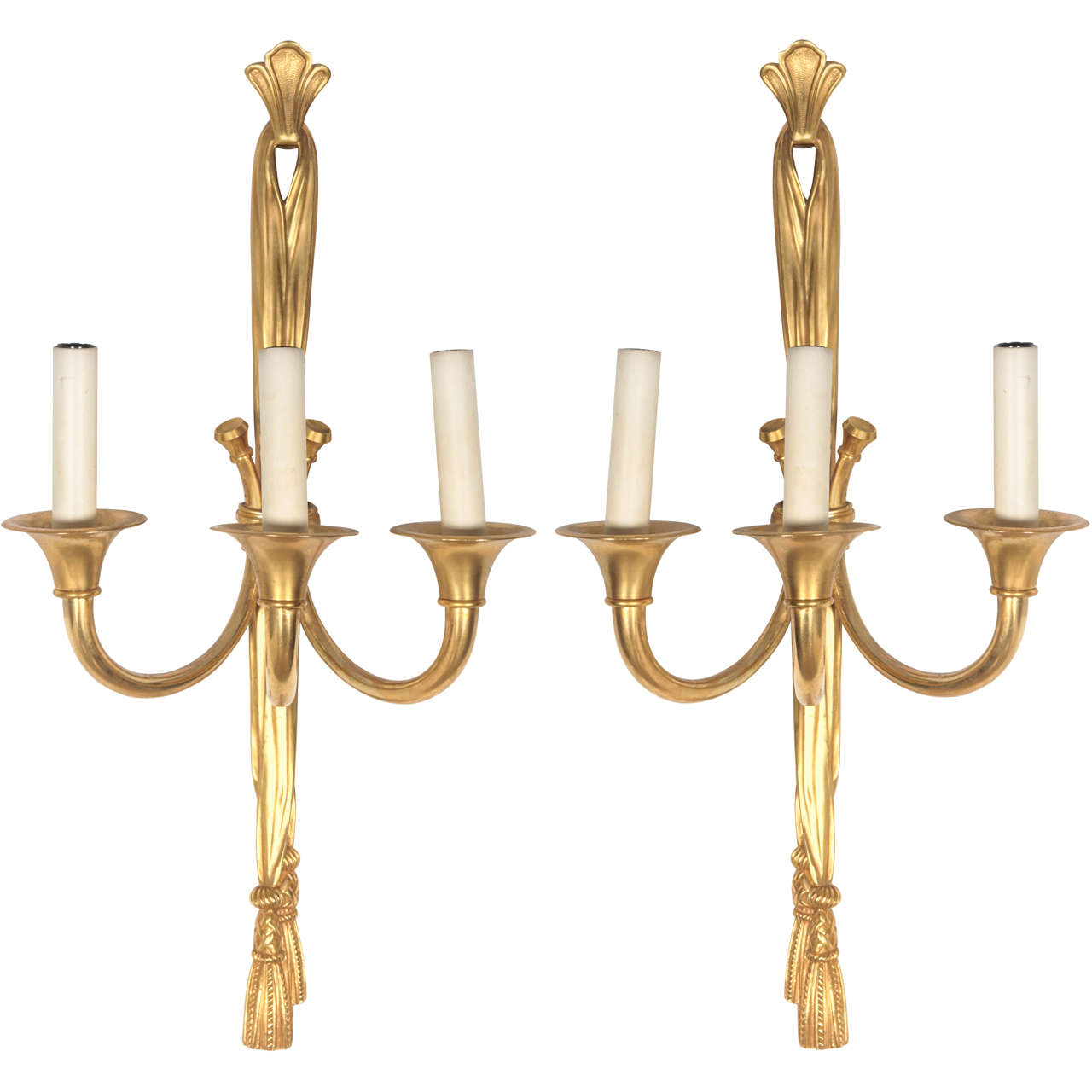This horizontal product photo showcases two large, ornate, gold wall sconces, set against a white background that creates the illusion they are floating in a void. Each sconce has a long, slender central beam adorned with decorative elements, culminating in gold tassels at the bottom. The sconces mirror each other at the base, with three gracefully curved, trumpet-shaped arms extending from the central beam, each ending in a white plastic cylinder designed to resemble a wax candle. These cylinders, which have small circular screws on top for light bulbs, are positioned to hold the electronic light fixtures. The overall design strikes an elegant, old-fashioned candle holder aesthetic. The sconces dominate the image, nearly filling the frame and centered prominently, lending an air of classical sophistication suitable for a high-end furniture catalog.